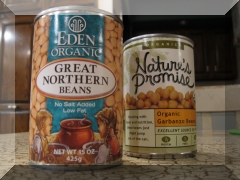The color photograph captures two cans of beans resting on a kitchen countertop that resembles marble, characterized by its white surface interspersed with gray streaks. On the left is a can of Eden Organic Great Northern Beans, which has a green label. The details on this can include a white oval with "Great Northern Beans" in black text surrounded by a light brown border. Below the oval, it states "No Salt Added" and "Low Fat" in white text. The can's imagery includes an illustration of a brown pot with beans, sitting beside two young children. The Nature's Promise can on the right features a design of lime green and white, with the brand name in black cursive. This can displays pictures of garbanzo beans and has several text blocks and logos, though some writing appears blurry. Additionally, it mentions "Organic" and "Excellent source" in black text within an orange rectangle. Both cans sit on the countertop, with a light brown cabinet and a black oven visible in the background.